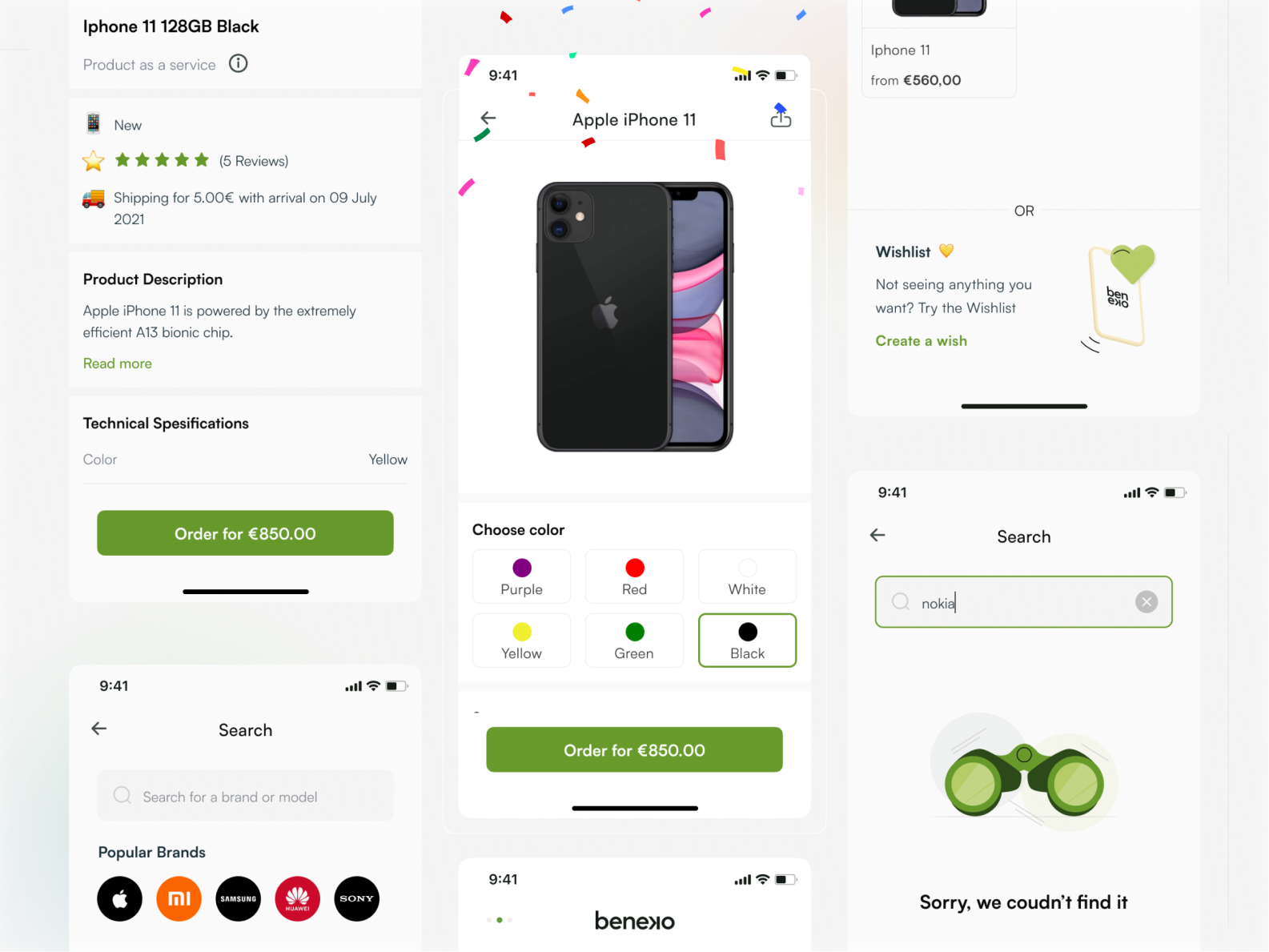**Product Listing: Apple iPhone 11 (128GB, Black)**

**Price:** $850  
**Condition:** New  
**Reviews:** 5 full star reviews  
**Shipping:** $5 (Estimated arrival: July 9, 2021)

**Product Description:** 
The Apple iPhone 11 boasts an efficient A13 Bionic chip, ensuring top-tier performance and power efficiency. Available technical specifications provide comprehensive details for tech enthusiasts.

**Available Colors:**  
- Black  
- Yellow  
- Purple  
- Red  
- Green  
- White  

**Additional Information:**  
- 941 bars of service  
- Wi-Fi enabled  
- Battery information  
- Easy search options for popular brands such as Apple, Samsung, and Sony  
- Order from $560, with wishlist options available for personalized tracking  

**Note:** Try utilizing the wishlist feature if the desired product is not immediately found. Make use of the search tool to filter by brand or model for more convenience.

**Availability:**  
Various models and colors are in stock, ready for immediate shipping.